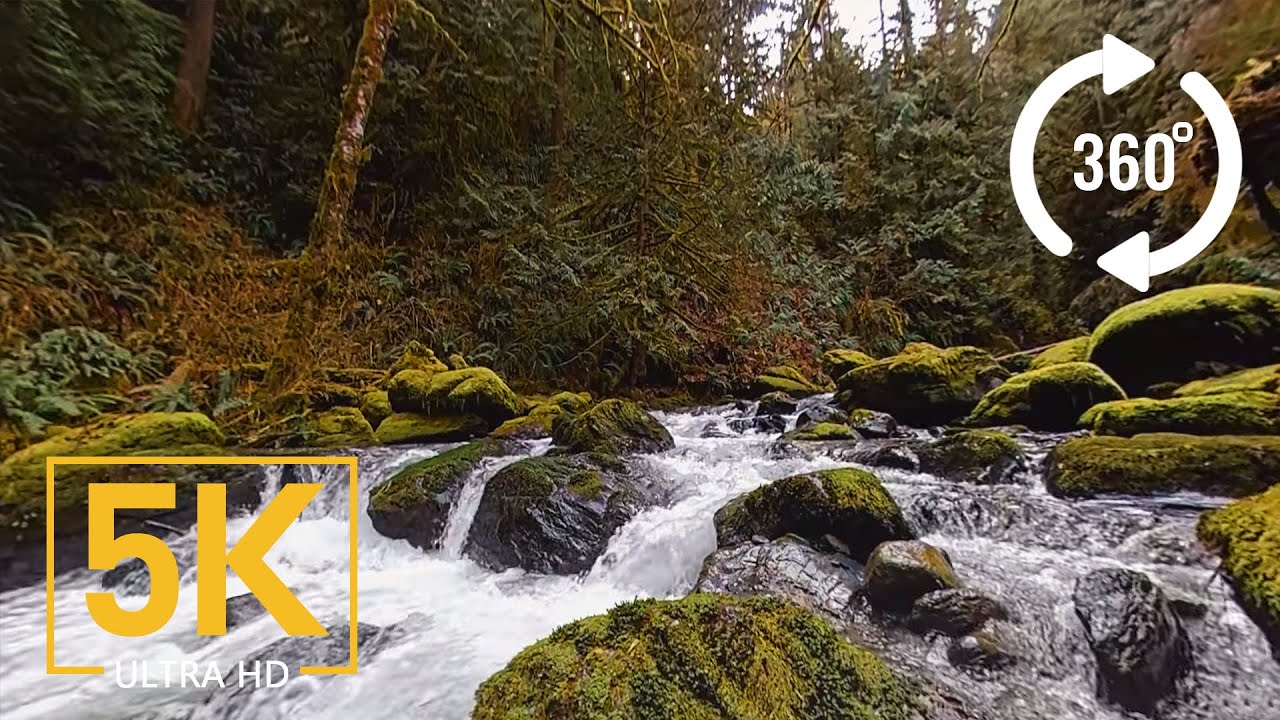The high-resolution photo captures an immersive, dynamic river or creek scene from the vantage point of standing in the river or right at its edge. Raging white water, in the form of rapids, rushes toward the camera, navigating over and around an array of large, moss-covered rocks that dot the river and its banks. The overall atmosphere is lush and verdant, with dense green foliage and tree trunks filling the background, extending onto a hill or mountain on the far side of the river. The vibrant greenery is punctuated by the occasional dead branch, adding a touch of natural complexity to the scene. On the photograph, the lower left corner features "5K Ultra HD" in bold yellow font within a yellow box, while the upper right corner displays "360 degrees" inside a circular arrow symbol, indicating the photo's panoramic, high-definition quality that invites viewers to look around as if they are present in the serene, verdant forest.